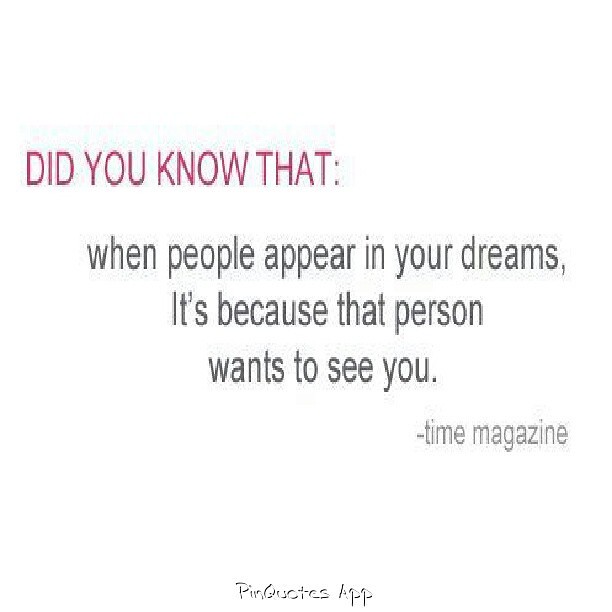The image is a grainy screen capture of a textual quote with a flat white background, possibly from a website or an app. At the top left, in large red, bold, all-caps letters, is the phrase "DID YOU KNOW THAT:". Below this, in black text, is the quote, "When people appear in your dreams, it's because that person wants to see you." The attribution "Time Magazine" appears underneath the quote in lighter gray font. At the very bottom, centered, the text "Pin Quotes App" is displayed in a basic, less bold print. There are no other images or elements in the picture.